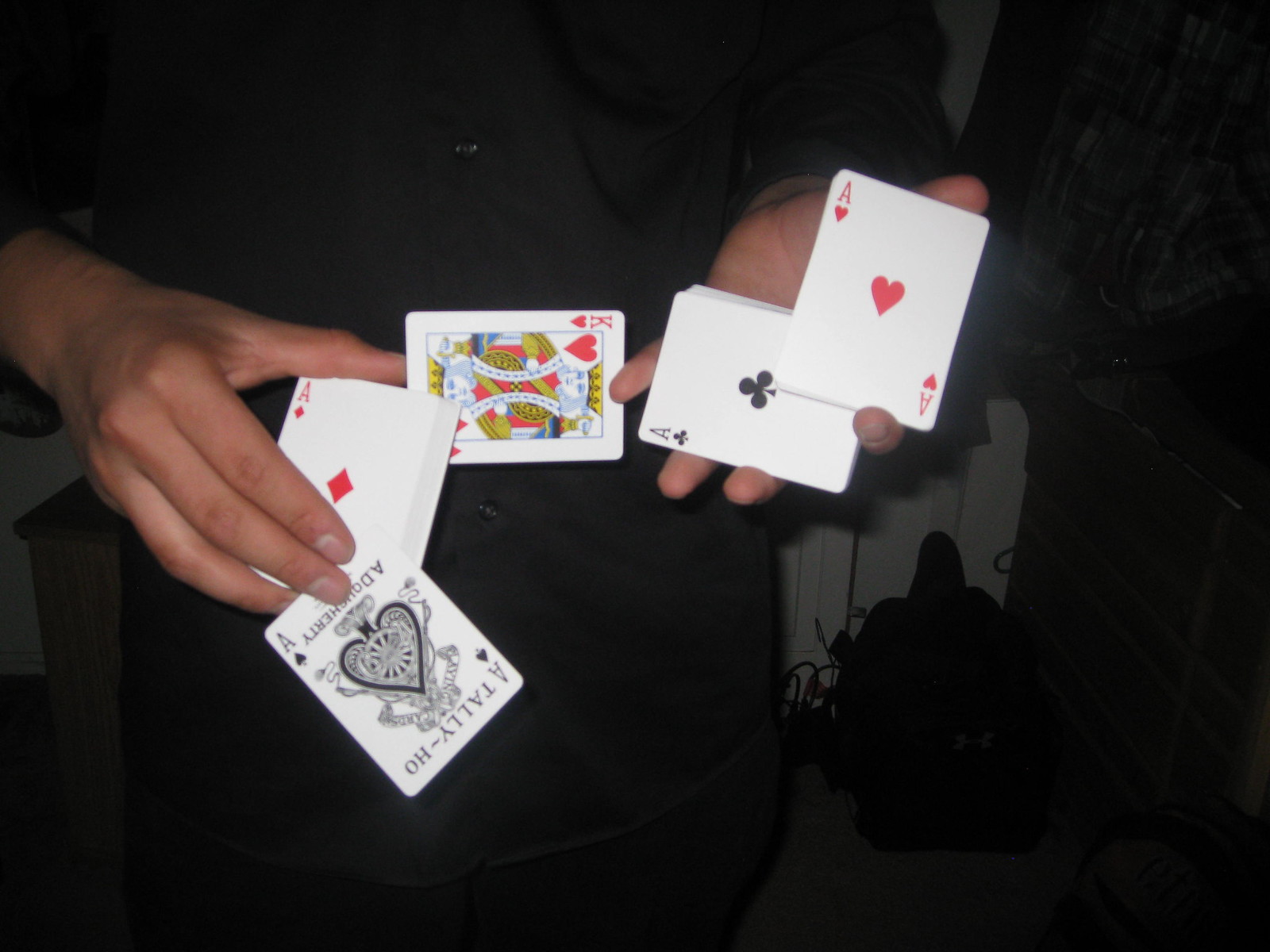In this photograph, a person dressed entirely in black is performing an intricate card trick. Only their hands and wrists are visible, drawing focus to the deck of cards they hold. The deck includes a prominently featured Ace of Spades from a Tally Ho card set, which showcases an elaborate spade design in the center and a distinctive logo at the bottom stating "A. Daughtry." Surrounding this card are other aces: the Ace of Diamonds in red, situated just above the Ace of Spades, and the Ace of Clubs, also horizontal, aligning with the King of Hearts which is positioned horizontally between both hands. The Ace of Hearts can be seen in the other hand, showcasing its vibrant red ink. The hands grip these cards skillfully, and there is an abundance of additional cards behind the Ace of Diamonds and Ace of Clubs, hinting at the complexity of the trick. A few other cards might be lurking behind the Ace of Hearts, but their numbers are uncertain. The composition highlights the vivid contrast between the red and black inks, emphasizing the magician's dexterity and the decorative elements of the Tally Ho card design.